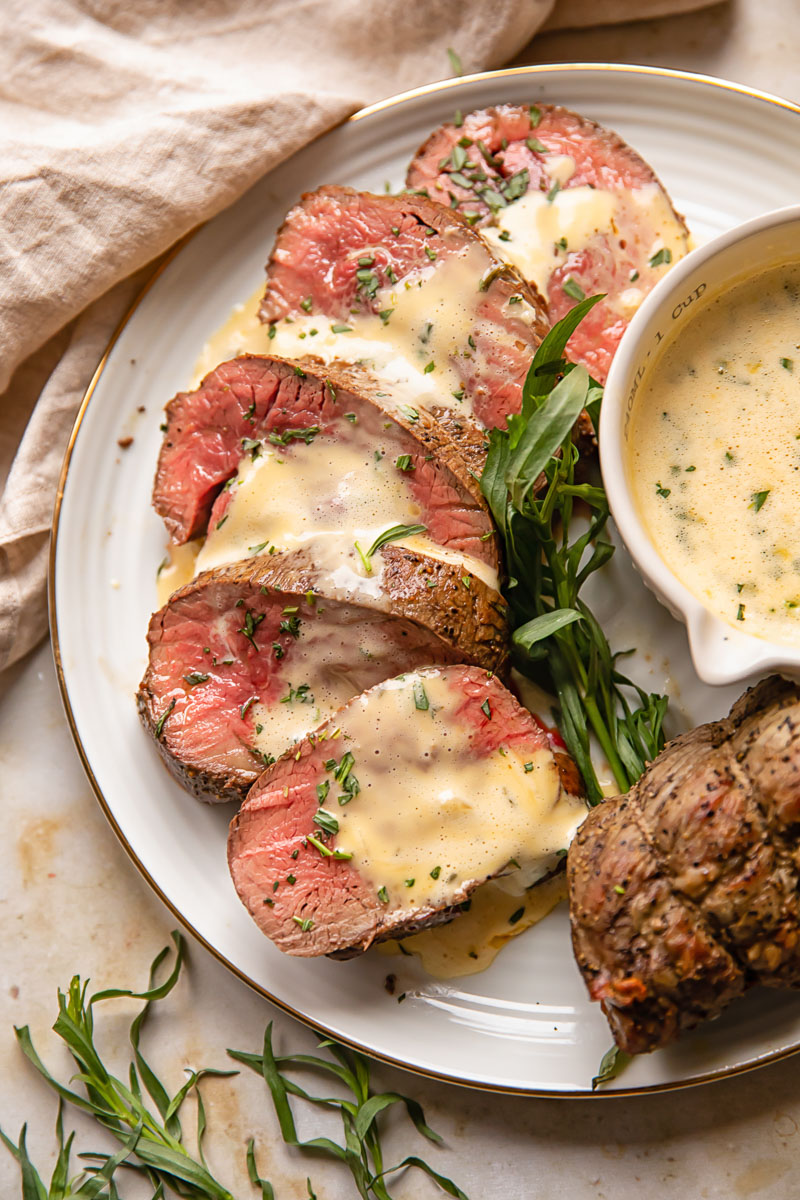The image displays a meticulously arranged indoor photographic scene from the vantage point of a person standing above a table setting. Central to the image is a white china plate adorned with a gold border, prominently featuring five rare, red slices of meat, each elliptical in shape and draped in a creamy yellow sauce. This rich sauce appears again in a small white bowl situated at the top-right corner of the plate, accompanied by a sprig of fresh green herbs. Below this bowl, a larger cut of meat suggests the origin of the sliced portions. The plate sits atop a beige tablecloth accented with green plants, while the upper portion of the image subtly includes a peach-colored napkin. Recurrent touches of green herbs pepper the display, adding a vibrant contrast to the overall earthy and rich tones of the presentation. No text accompanies the image.